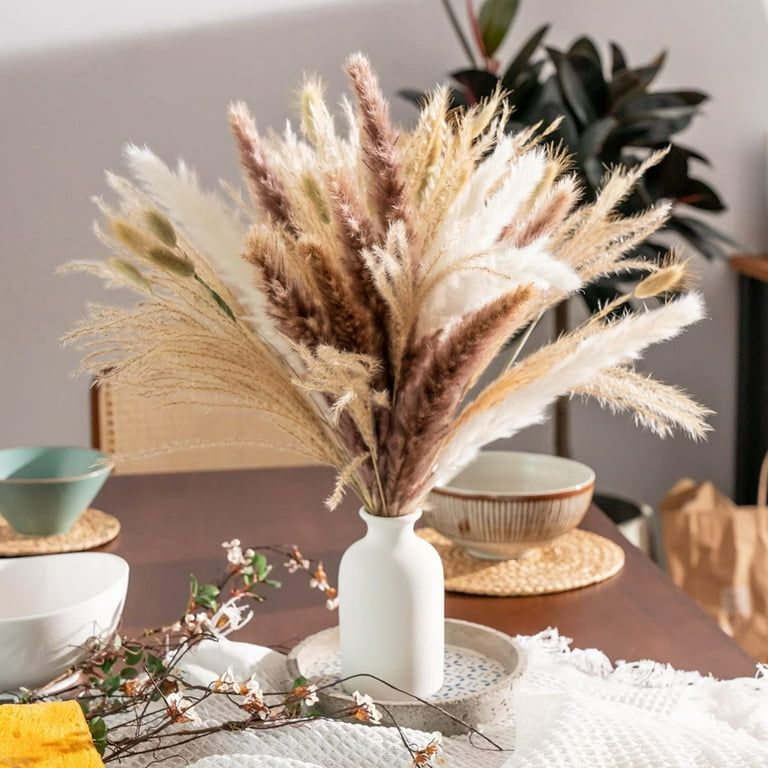This square-format color photograph, taken indoors, captures an artfully arranged tabletop decor on a light mauve dining table. Dominating the center is a white vase with rounded corners and a flared top, filled with a bouquet of dried stalks, cattails, golden wheat stems, and various beige and brown flowers, which fan out like a feather headdress. The table is decorated with various vessels: to the right, a round ceramic bowl with vertical brown stripes sits on a woven, basket-like coaster, and to the left, an aqua ceramic dish rests on a similar coaster. In the lower left corner, a white ceramic dish and a sprig of wildflowers are placed near a yellow sponge adorned with wire strands and small pink and green flowers. A fringed white tablecloth underlies the entire arrangement. The background features a white wall with a dark green plant and a chair, adding depth to the scene. The overall style of the photograph is representational realism, capturing the fine details and textures of each element.